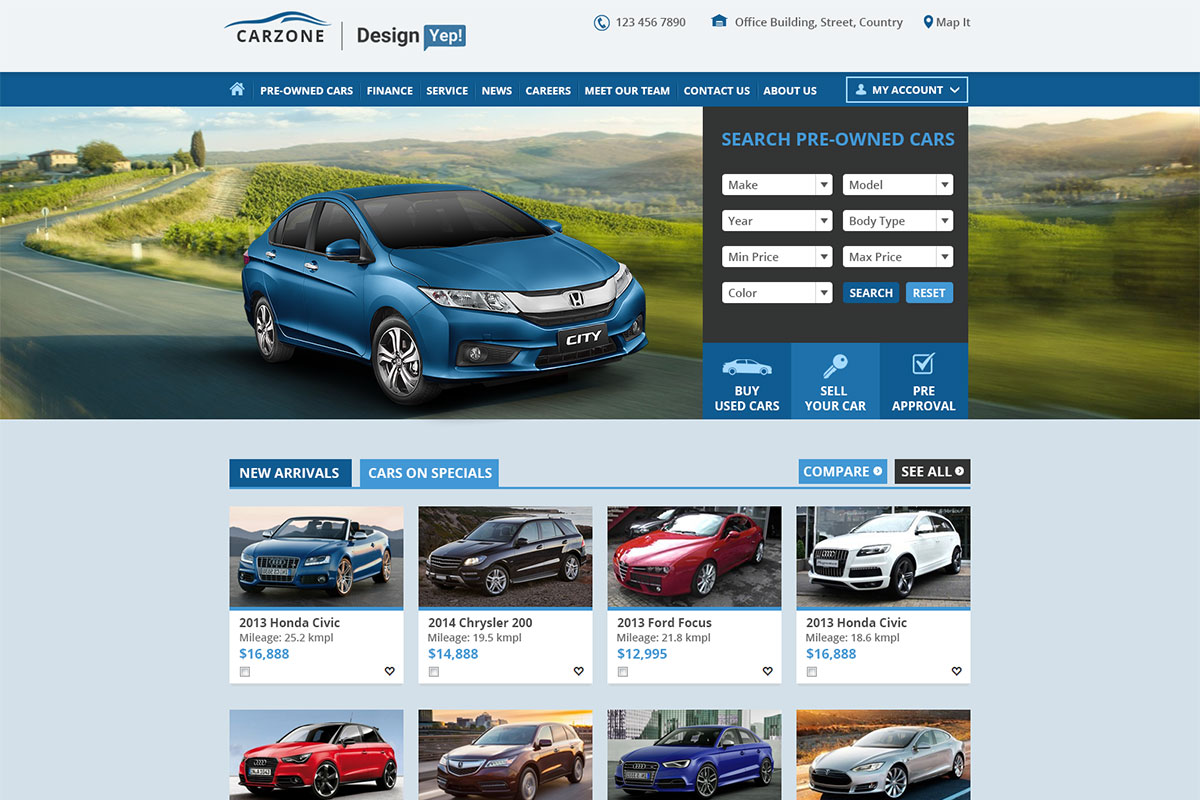The provided image is a detailed screenshot of a website's homepage, presented in a landscape orientation which makes it wider than it is tall. At the very top of the page, there is a slim, light blue strip featuring the logo and name "Car Zone." The logo includes an abstract depiction of a small, bluish hill. Adjacent to the logo, the word "Design" is visible, along with a small blue speech bubble containing the word "Yep" in white text.

Further down, the website prominently displays a WhatsApp contact number: 123-456-7890, situated next to an icon of a house accompanied by "Office Building, Street, Country" - possibly indicating a placeholder for a physical address.

Beneath this, there is a prominent navy blue navigation bar with multiple menu options including: "Pre-Owned Cars," "Finance," "Service," "News," "Careers," "Meet Our Team," "Contact Us," "About Us," and a drop-down menu labeled "My Account."

Dominating the main section of the page is a rendering of a sleek blue sedan driving along a picturesque country road. The backdrop of this image showcases mountains and green fields under a daylight sky, adding a serene visual appeal. 

To the right of the car rendering, a search box is available for users to find pre-owned cars. It includes drop-down options for specifying make, model, year, body type, minimum price, maximum price, and color. Two blue buttons labeled "Search" and "Reset" accompany the search fields.

At the bottom of the page, there are three blue boxes with white text offering additional services: "Buy Used Cars," "Sell Your Car," and "Pre-Approval." Below the main image and search box area, there's a larger light blue section displaying various car listings, such as a 2013 Honda Civic and a 2014 Chrysler 200. 

Overall, the image portrays a thoughtfully designed car dealership website with user-friendly navigation and comprehensive search functionalities to assist potential customers in their car buying journey.